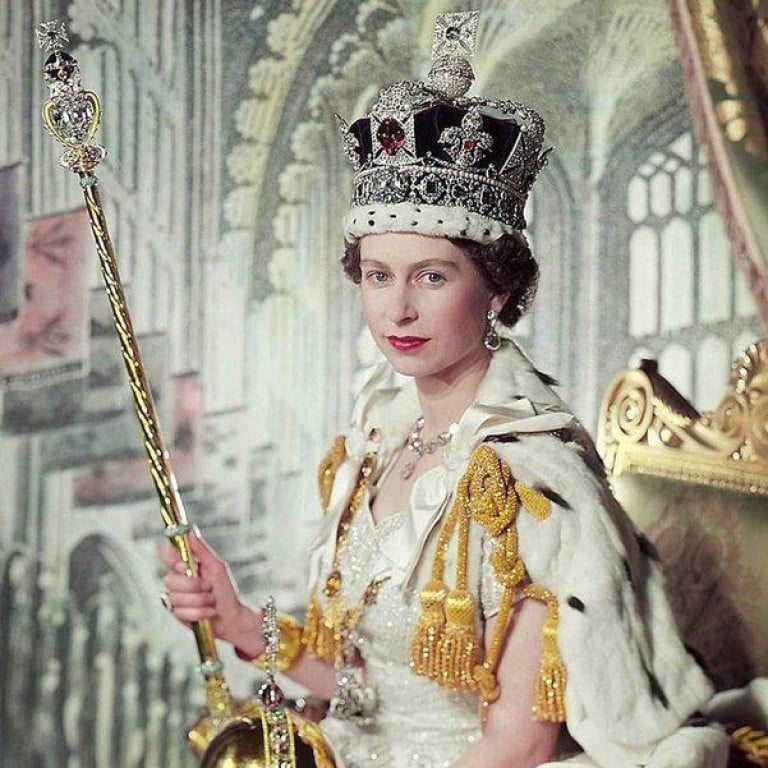The photograph features a regal-looking woman, who appears to be a queen, seated on an opulent golden chair. She is wearing an elaborate maroon crown adorned with silver details and gems, and it is bordered at the base with white fur dotted with black spots. Her brown, curly hair cascades elegantly, and she dons pink lipstick which enhances her royal appearance. She is enveloped in a long, white fur cape, also featuring black spots, and beneath it, she wears a sparkly, glittery white dress decorated with gold tassels that hang from ropes on either side. In her right arm, bent at the elbow, she holds a baton that is topped with a cross. The backdrop suggests she is in a grand, possibly historic, setting with towering walls that emphasize the magnificence of her surroundings. Her attire and the setting evoke imagery of historical or cinematic portrayals of royalty.